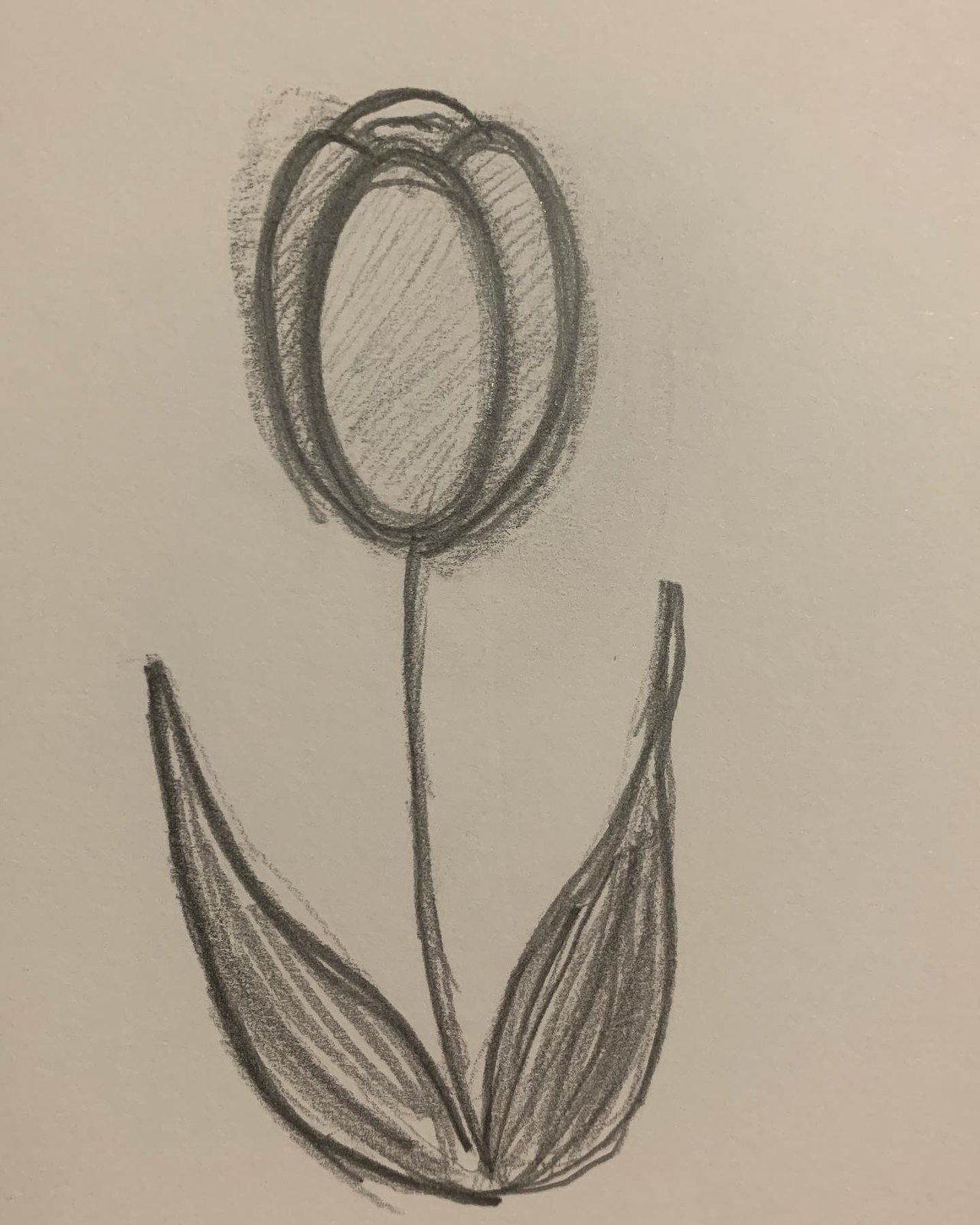A pencil drawing of a flower, likely a tulip, graces a sheet of light lilac-colored paper. The center features a carefully drawn stem, flanked by two leaves angled upward. The edges of these leaves are subtly darkened with pencil strokes, and their interiors are textured with soft, side-of-pencil shading. At the stem's pinnacle blooms the tulip, characterized by its four distinct petal sections. One prominent oval petal occupies the foreground, accompanied by two partial ovals on either side and a small arc suggesting the rear petal. The flower's interior hints at its stamen, shaded diagonally to add depth and realism.